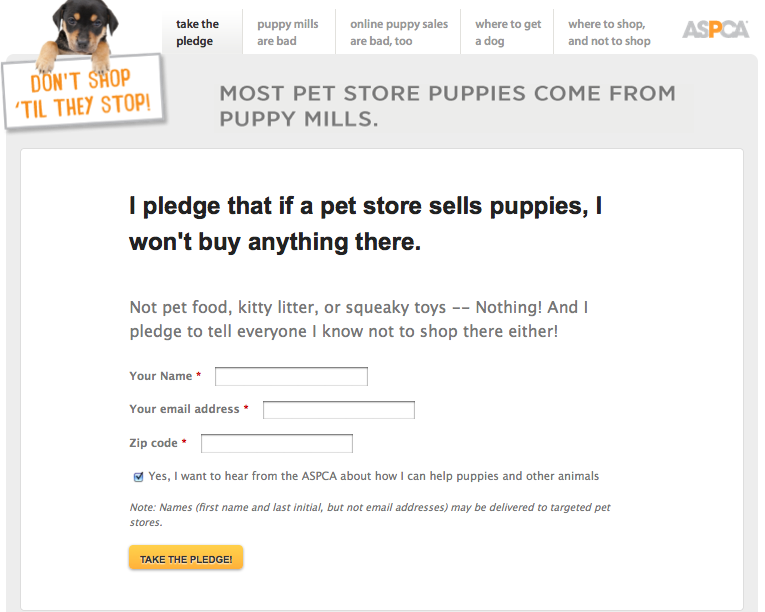The image is a detailed screenshot of the ASPCA website. At the top right, prominently displayed, is the ASPCA logo. Below the logo, there are several navigational categories including "Take the Pledge," "Puppy Mills are Bad," "Online Puppy Sales are Bad Too," "Where to Get a Dog," and "Where to Shop and Not to Shop." 

To the left of these categories is an image of a puppy holding a sign that reads, "Don't Shop Till They Stop." Below the puppy, there is a bold statement: "Most pet store puppies come from puppy mills." 

Further down, a pledge is outlined for site visitors: "I pledge that if a pet store sells puppies, I won't buy anything there—not pet food, kitty litter, or squeaky toys. Nothing. I pledge to tell everyone I know not to shop there either." 

Towards the bottom of the page, there are text boxes prompting visitors to input their name, email address, and zip code. Additionally, there's a checkbox labeled, "Yes, I want to hear from the ASPCA about how I can help puppies and other animals."